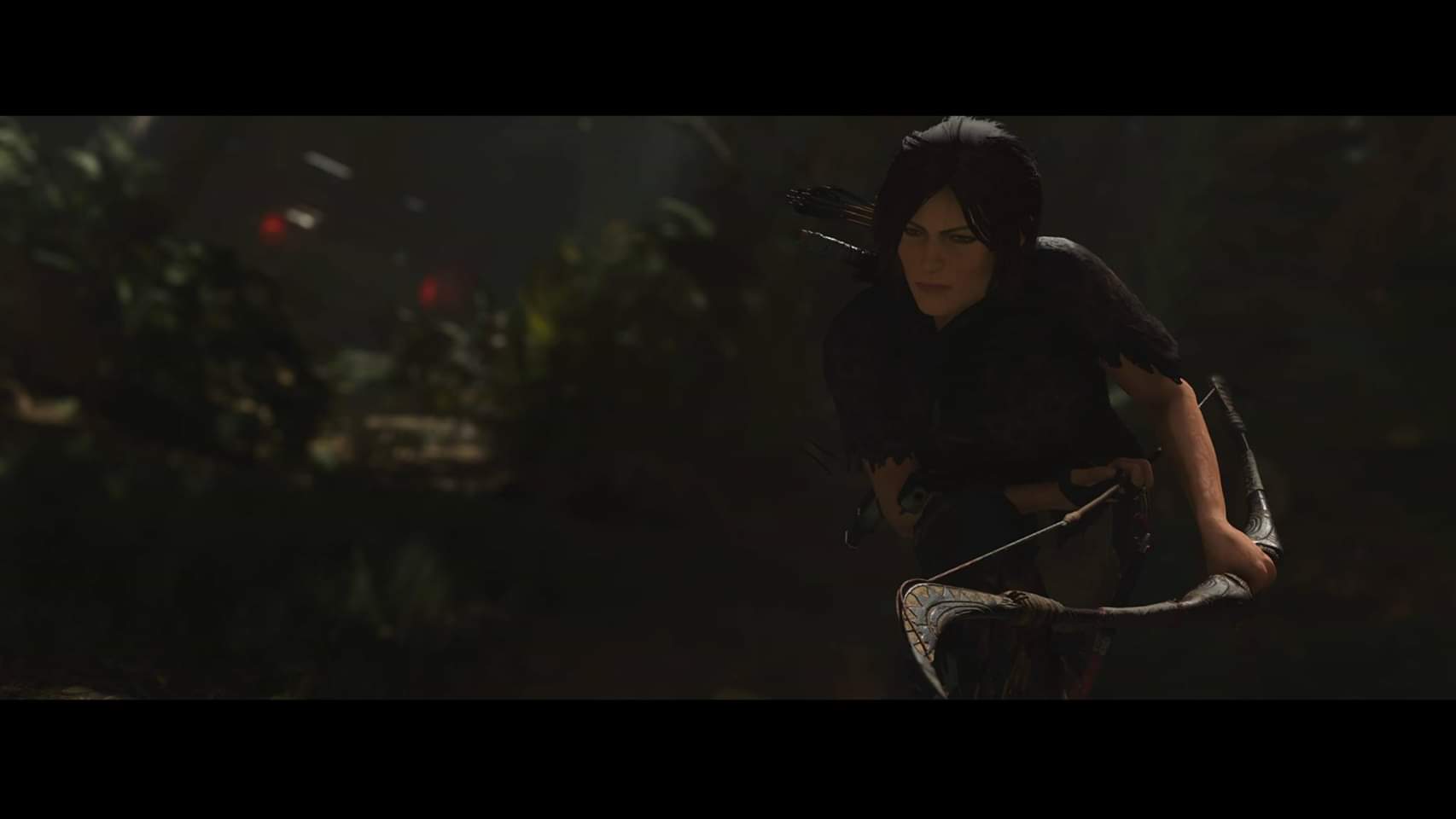A screenshot from a 3D video game depicts a dark, hazy background that lends a mysterious ambiance to the scene. On the left side, jagged green foliage forms a noticeable point and features two conspicuous red dots. To the right, a woman is captured mid-run, gripping a bow under her arm. With her right hand, she holds the string, while her left hand steadies the bow at its midpoint. Quivers of arrows are visible protruding from behind her back. She is dressed in a brown shirt with ragged, torn-off sleeves, adding to the rugged nature of her character.